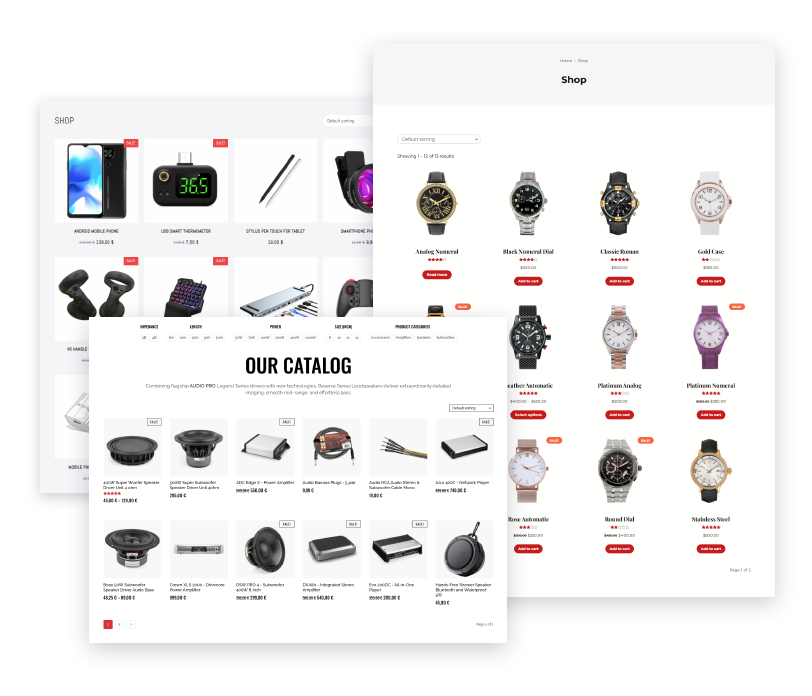The image is a composite screenshot of what appears to be a watch catalogue. It consists of three different sections merged together:

1. **Top Left Section - "Our Catalogue"**: This part primarily showcases various computer accessories. The items displayed include peripherals or add-ons that might be used alongside a computer setup.

2. **Top Right Section - "Shop"**: This section is dedicated to a collection of watches. It features an assortment of watch designs and styles, indicating a focus on timepieces available for purchase.

3. **Bottom Left Section - Partially Hidden "Shop"**: This section seems slightly obscured but indicates a diverse range of products. It includes visuals of a phone, an alarm clock, a stylus, and items resembling VR controllers or handles, suggesting it encompasses a variety of tech gadgets and accessories.

The image creates a cohesive view of different product categories available in the catalogue, from computer accessories to watches and other tech gadgets.